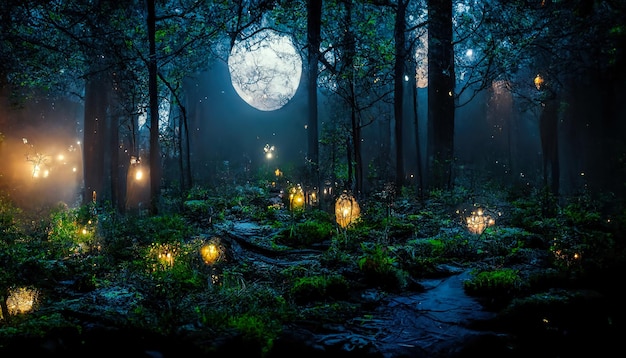The image portrays a scene of a nighttime forest that exudes a magical, perhaps computer-generated vibe. Tall, thin tree trunks rise into the night sky, their sparse branches allowing glimpses of a massive, bright moon positioned in the background. This celestial body, with its unusual size and lack of perfect circularity, casts doubt on its authenticity, perhaps signaling another light source or artistic embellishment. 

On the ground, a meandering path is softly illuminated by numerous lanterns or fairy lights, their warm, yellow glow interspersed with specks of light reminiscent of fireflies. Shrubs and dark green, lush but low-lying bushes punctuate the scene, along with what appears to be wet soil or glistening water, enhancing the mystical atmosphere. 

To the far right, a suggestive figure, possibly a deformed tree, holds up yet another glowing light, adding to the enigmatic feel. Meanwhile, a hazy, smoggy patch on the left further contributes to the ethereal mood. With no stars visible, the image relies on these scattered light sources to create an enchanting, almost surreal forest landscape.